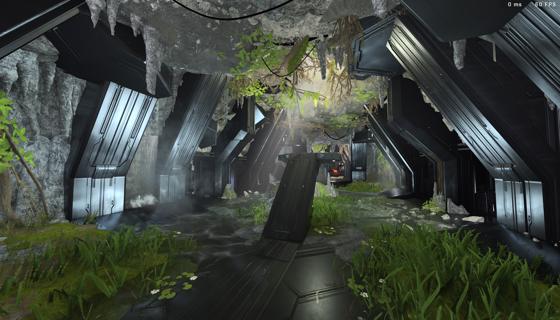The image showcases a futuristic scene set against a gray, overcast sky with touches of white, perhaps clouds or light diffusion. Dominating the landscape are towering metal structures that extend downwards from the sky. These structures, predominantly gray, vary in shape with some exhibiting bends and joints, adding an abstract, almost surreal quality to the scene. The foreground features a metallic stairway alongside a large, slanted piece of metal, contributing to the industrial aesthetic. The environment is softened by a yard of green grass dotted with small white flowers. A metal walkway, consistent with the metallic theme, cuts through the yard. The scene is partially framed by overhanging tree branches, and jagged metal pieces are seen hanging over a nearby fence, enhancing the juxtaposition of nature and industry.